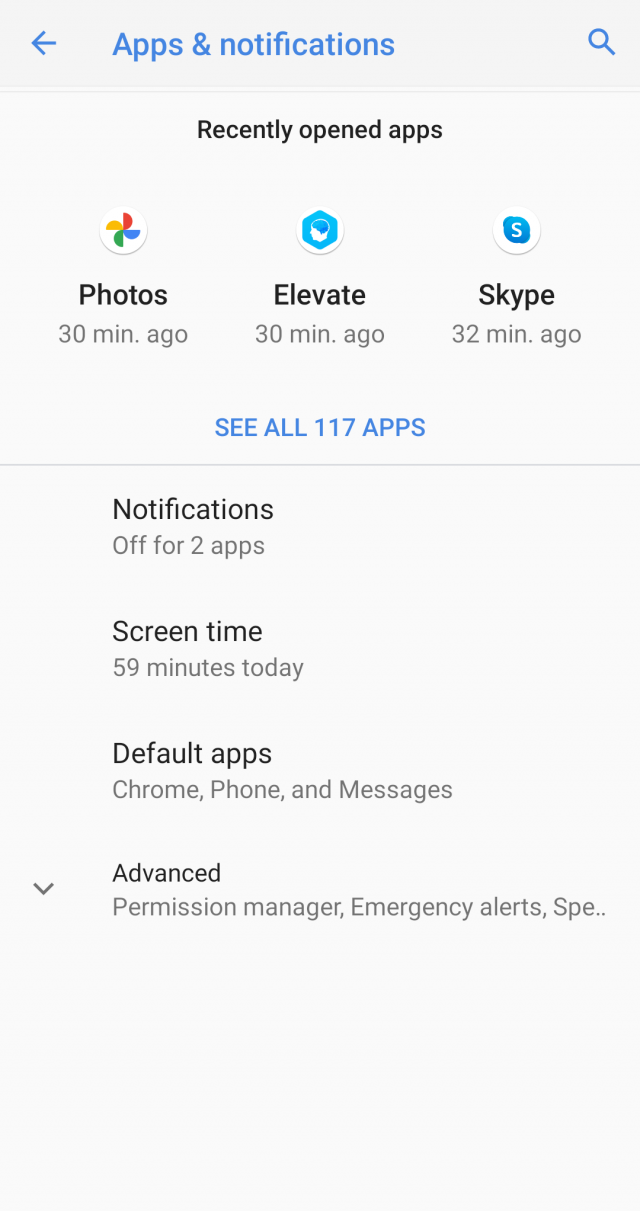The top section of the screenshot features a light gray background. On the left side, a blue arrow points to the left, alongside the word "Apps" in blue, with a capital 'A'. To the right of "Apps," there's a blue magnifying glass icon. Two thin gray lines run horizontally across the screen underneath this section.

Below these lines, the background turns gray. In the middle, the text "Recently Open Apps" appears in black, with both 'R' and 'O' capitalized. There are three circular icons lined up vertically beneath this heading:

1. The first circle contains a mix of red, yellow, green, and blue colors. Below this circle, the word "Photos" appears in black text, followed by "30MIN.AGO" in gray text.
2. The second circle features a blue hexagon. Below it, "Elevate" is written in black, with "30MIN.AGO" in gray text underneath.
3. The third circle, displaying a blue background with a white 'S' in the center, represents Skype. Below it, "Skype" is written in black, with "32MIN.AGO" in gray text.

Further down, in all capital letters and blue text, the phrase "See all 117 Apps" is displayed. Another thin gray line runs horizontally below this.

Next, the text "Notification" appears in black. Below this, "All for 2 Apps" is written in gray.

After some space, the following information appears:

- "Screen Time" in black, followed by "59 Minutes Today" in gray.
- "Default Apps" in black, with "Chrome, Phone, and Messages" in gray underneath.
- "Advanced" in black, with "Permission Manager, Emergency Alerts, SPE" written in gray below, followed by an ellipsis ("...").

The viewable portion of the screenshot ends here.